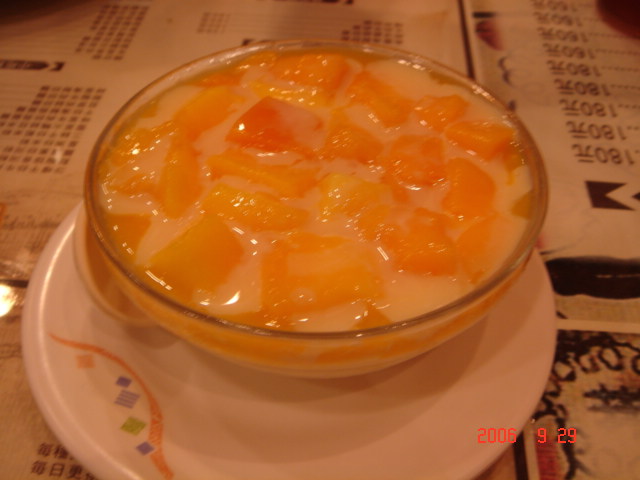In this image, we observe a close-up of a glass bowl filled with chunks of orange-yellow fruit, possibly peaches, immersed in a white liquid that may be milk or yogurt. The bowl is positioned in the center of the image and rests on a thin white plate, which features a small orange design in the left-hand corner. The setting appears to be a restaurant, as evidenced by the menus or paper tablecloth partially visible on the table beneath. The table displays some glare, adding to the ambiance. The colors present in the image include white, orange, yellow, purple, green, black, gray, and red. Notably, the date "2006 929" is clearly visible in orange letters in the bottom right corner. The overall scene suggests a meal setting characterized by a mixture of cultural or regional elements, implied by the unreadable foreign text on the menus.